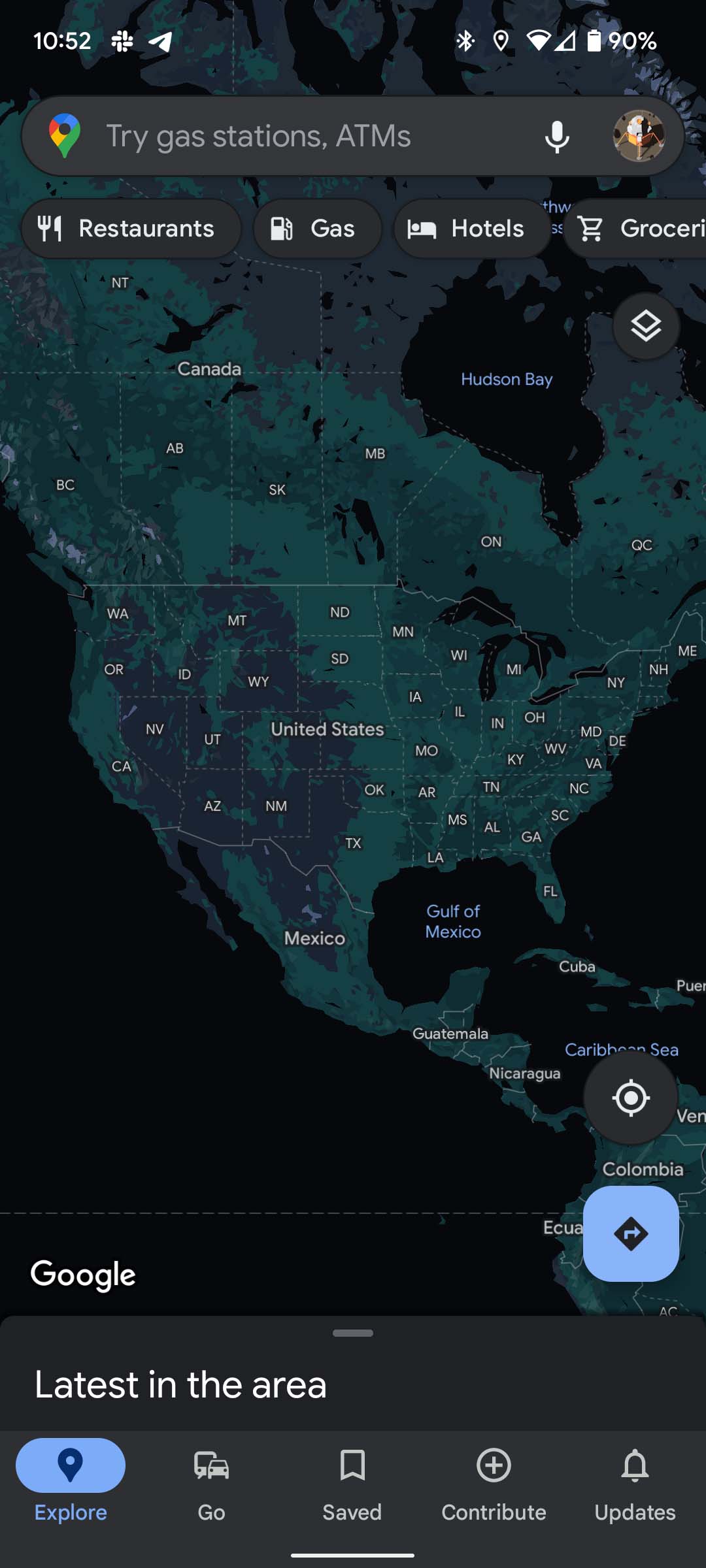This is a detailed screenshot from a mobile phone displaying various elements on its screen. At the topmost part of the screen, in white font, information about the phone is shown. Starting from the left, it indicates the time as 10:52, followed by a sequence of icons: a cross icon, a location sharing icon, a Bluetooth icon, a mobile signal icon, a Wi-Fi signal icon, and a battery icon displaying 90% charge at the far right.

Immediately beneath this information is a map covering the continental USA, Canada, and Central America. The ocean areas on the map are depicted in black, while the landmasses are shown in dark grayscale tones. At the top of the map, there's a gray oval search field. On the left side of this field is a rainbow-colored location sharing arrow, suggesting the use of Google services.

Within the search field, the placeholder text reads "Try gas stations, ATMs." To the right of this text are a white microphone icon and a small profile picture, which is too small to discern any details.

Positioned below the search field are four gray bubbles with text, each representing quick access categories: "Restaurants," "Gas," "Hotels," and "Groceries."